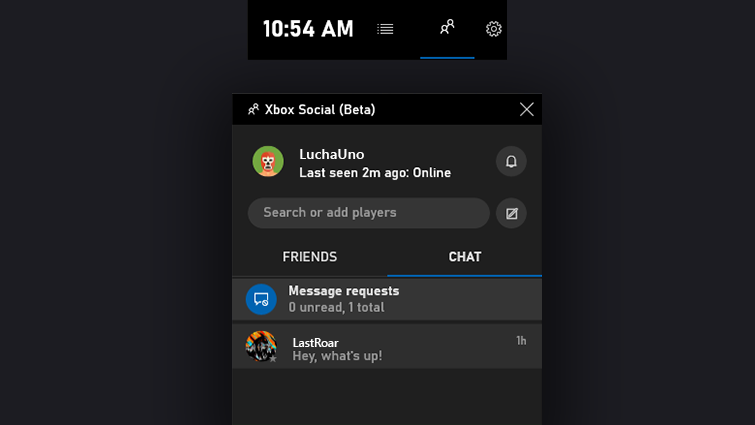The image showcases a dark-themed interface, typical of a gaming console's social screen. At the top left, the time is displayed as **10:54 AM** alongside a **settings button**. Beneath the header, bold text reads **"Xbox Social"** with **"(Beta)"** in parentheses. 

To the top right, there is an **X** button for closing the screen. 

The main content features a list of friends and status updates. One friend, **Lucha Uno**, was last seen **two minutes ago**, indicated as **online**. An avatar representing Lucha Uno is depicted with a **red mask and white face paint**, resembling a clown, set on a **green background**. Next to Lucha Uno's status, there is a clickable **notification bell** icon. 

Below the friends' statuses, there is a **search field** labeled **"search or add players"**, along with sections for **Friends** and **Chat**. 

Under the Chat section, it states there are **zero unread and one total** message requests. The only message visible is from **Last Roar**, stating **"hey, what's up?"** received **one hour ago**. Last Roar's avatar features a character with **black hair** on an **orange background** with other colors.

The interface is predominantly **dark gray or black**, commonly seen on gaming screens, enhancing the vividness of the avatars and text.